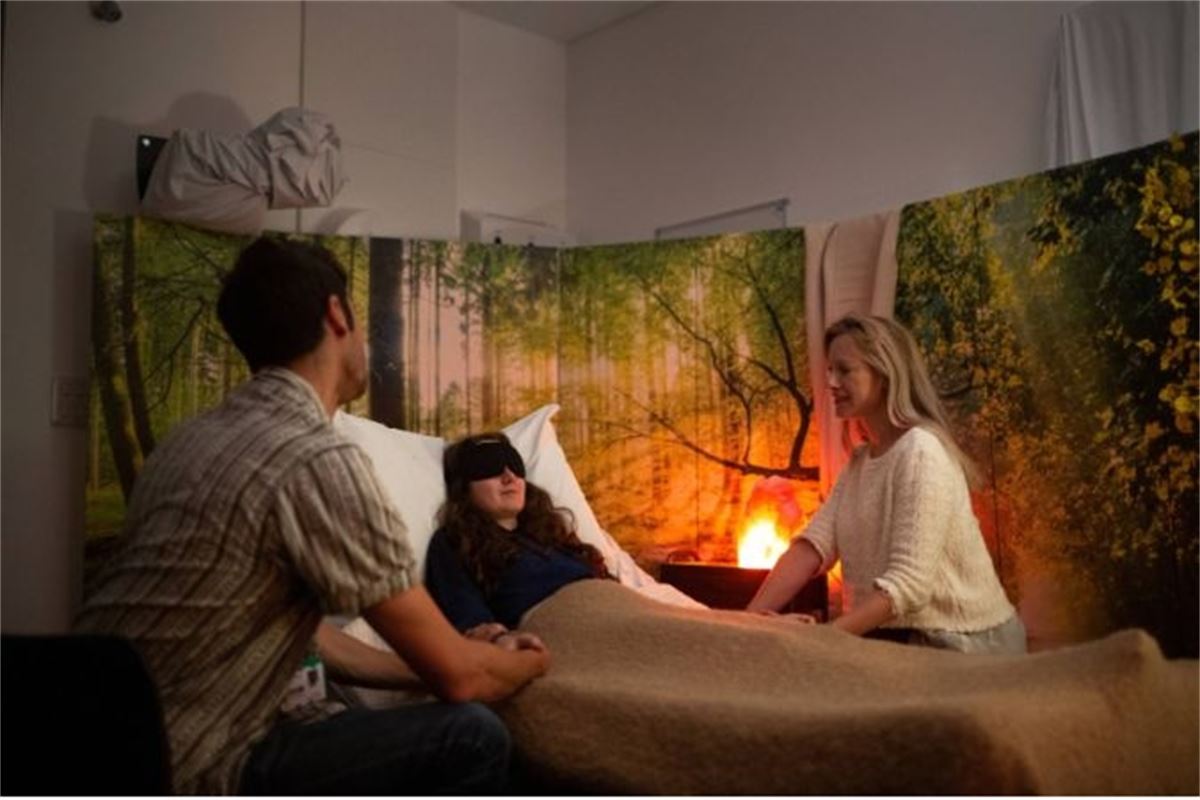In the center of a warmly-lit, white room, a young woman with long brown hair is lying in a bed, possibly a hospital bed, and is visibly propped up against several white pillows. A tan or brown blanket covers her up to her waist, and she is wearing a black sleep mask over her eyes. On either side of her, a man and a woman, possibly her parents, are seated and holding her hands. The man, dressed in a brown and white striped short-sleeved shirt and jeans, sits on the left side of the image with his back to the camera. The woman, with blonde hair, wears a white sweater and gray pants and sits on the right side of the image, smiling at the young woman. Behind the bed, a tapestry with images of a forest scene, presumably covering lights or windows, adds a nature-inspired backdrop that is softly illuminated, giving the room a warm, campfire-like glow.